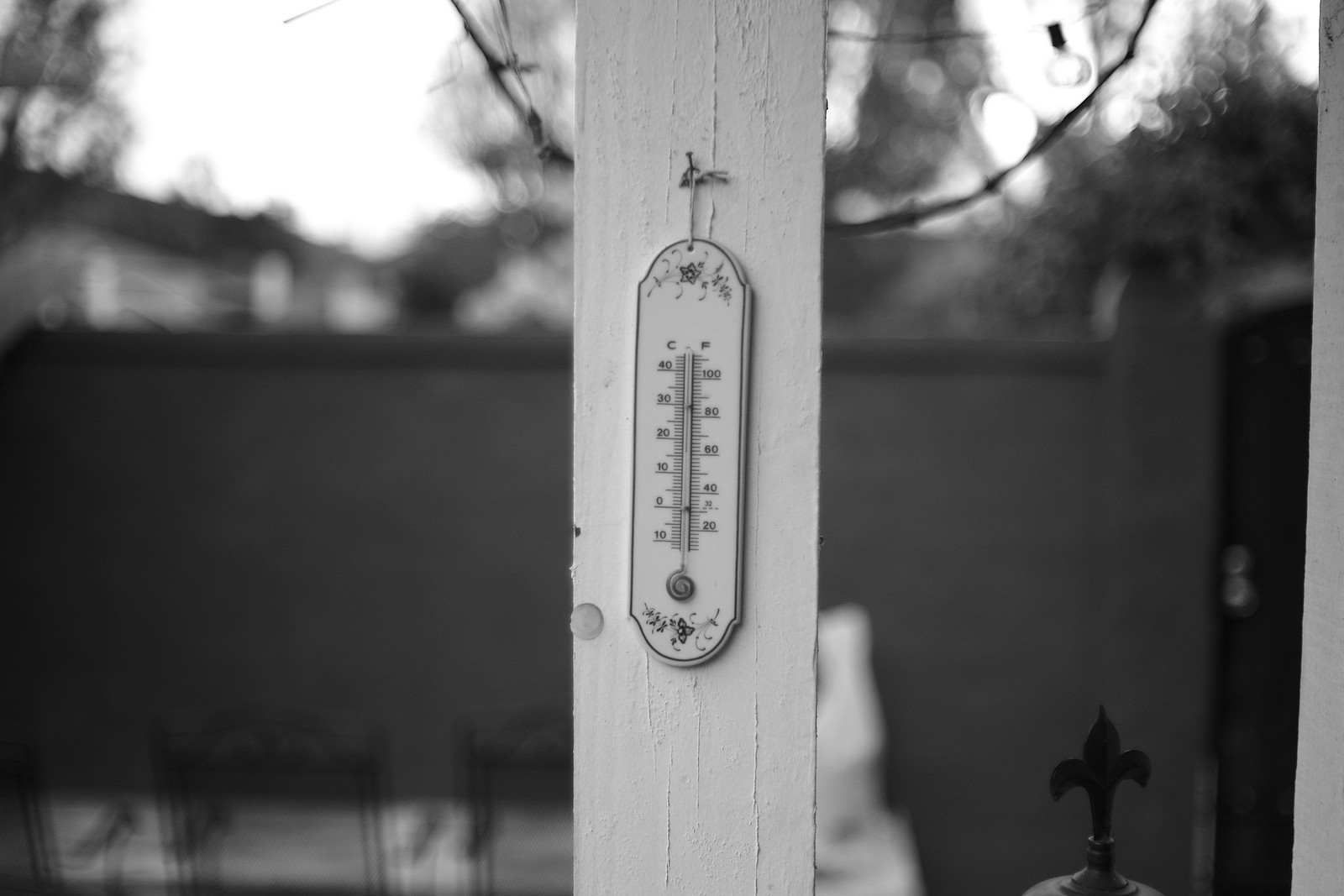In this black and white photograph, we find ourselves in a serene backyard or patio setting. The scene is anchored by a long wall that seems to serve as a boundary, likely separating this yard from the neighboring house that can be vaguely discerned in the blurred background. The foreground reveals a cozy arrangement featuring three chairs, suggestive of a patio setting, and likely indicating the presence of a table.

Attention is drawn towards the right side of the image where we see a door, perhaps leading to the driveway or offering access to another part of the house. Central to the composition is a white-painted column, its paint slightly peeling, adding a touch of rustic charm. Affixed to this column is a small, cylindrical thermometer, approximately six inches in length. This thermometer, marked with readings for both Celsius and Fahrenheit, shows temperatures ranging from 0 to 40 degrees Celsius and 0 to 100 degrees Fahrenheit. Currently, the temperature reads approximately 82 degrees Fahrenheit (29 degrees Celsius), with corresponding markers for critical temperatures such as 0 and 32 degrees Fahrenheit.

The thermometer itself is a quaint piece, adorned with intricate floral designs at its top and bottom, and a delicate swirl pattern in the center, all adding a touch of elegance to this functional item. The scene perfectly captures a moment of quiet observation in a domestic setting, filled with subtle details that hint at the everyday life and character of the space.